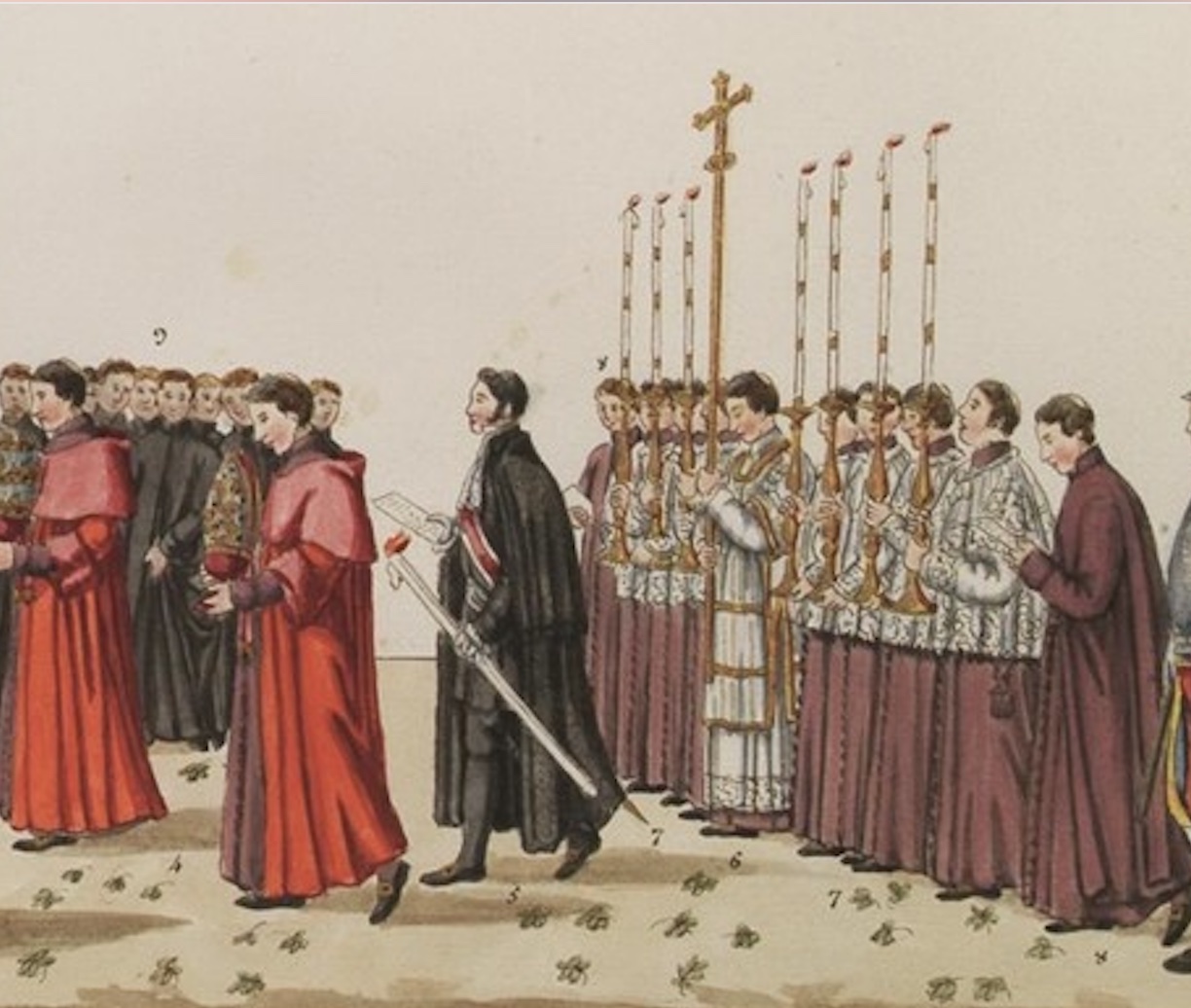This detailed artwork, likely created around the 1800s, depicts a ceremonial religious service set indoors, with the time of day uncertain. The scene is filled with rows of people, primarily focused on the right-hand side. In the background, a line of men dressed in plum-colored robes that reach their feet is holding various ceremonial objects, including a large gold cross and long, gold-like staffs. Leading this line, a young man in a long black robe, adorned with a cape, carries a long, white staff or sword in his left hand. In front of him, other participants are dressed in an array of colors such as red, brown, light maroon, and dark green. Some of these men in red and black robes are scattered throughout the composition, with a group situated in the top left corner and others meandering about, all facing towards the right. The cohesive use of colors, traditional attire, and religious artifacts vividly convey the solemnity and ritualistic nature of the depicted ceremony.